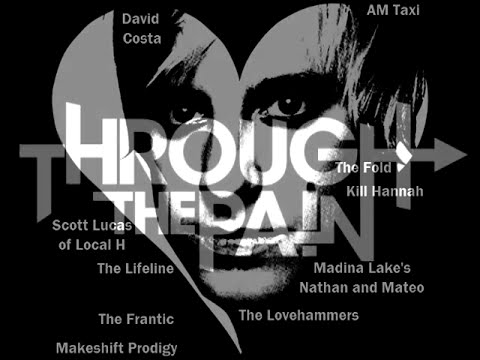The image features a monochromatic palette of black, white, and gray. Dominating the composition is a heart shape at the center, containing the silhouette of a man’s face with dark eyes and a closed mouth. Prominently displayed in the middle of the image is the text "Through the Pain," with a distinctive white arrow piercing through the "H." Additional text clustered around this focal point includes "The Fold" and "Kill Hannah." 

Positioned in the top left corner is the name "David Costa," while the top right features "A.M. Taxi." Below the central text, on the left side, various names cascade downwards: "Scott Lucas of Local H," "The Lifeline," "The Frantic," and "Makeshift Prodigy." Meanwhile, the bottom right corner lists "Medina Lake’s Nathan and Mateo" and "The Love Hammers." 

The entirety of the text and imagery is rendered in stark white against the black background, suggesting it might be an advertisement or poster for a music event, possibly highlighting various alternative rock bands.